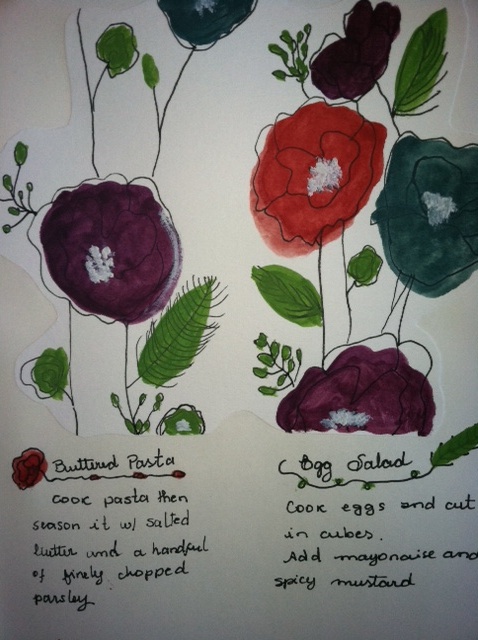The photograph captures a vibrant collage featuring roughly sketched, brightly colored flowers cut from a piece of white paper and pasted onto an off-white wall. The flowers—purple, red, and bluish-green—have been colored with markers, intentionally spilling outside the lines to create a casual, whimsical aesthetic. Each flower showcases a white center, with stems and leaves drawn in the same freehand style. Below the floral artwork, written directly on the wall with what appears to be a Sharpie, are recipes for 'Buttered Pasta' and 'Egg Salad.' The 'Buttered Pasta' recipe instructs to cook pasta, then season it with salted butter and a handful of finely chopped parsley. Adjacent to it, the 'Egg Salad' recipe advises cooking eggs, cutting them into cubes, and mixing them with mayonnaise and spicy mustard. These handwritten instructions add a practical touch to the decorative display, combining culinary tips with artistic expression.